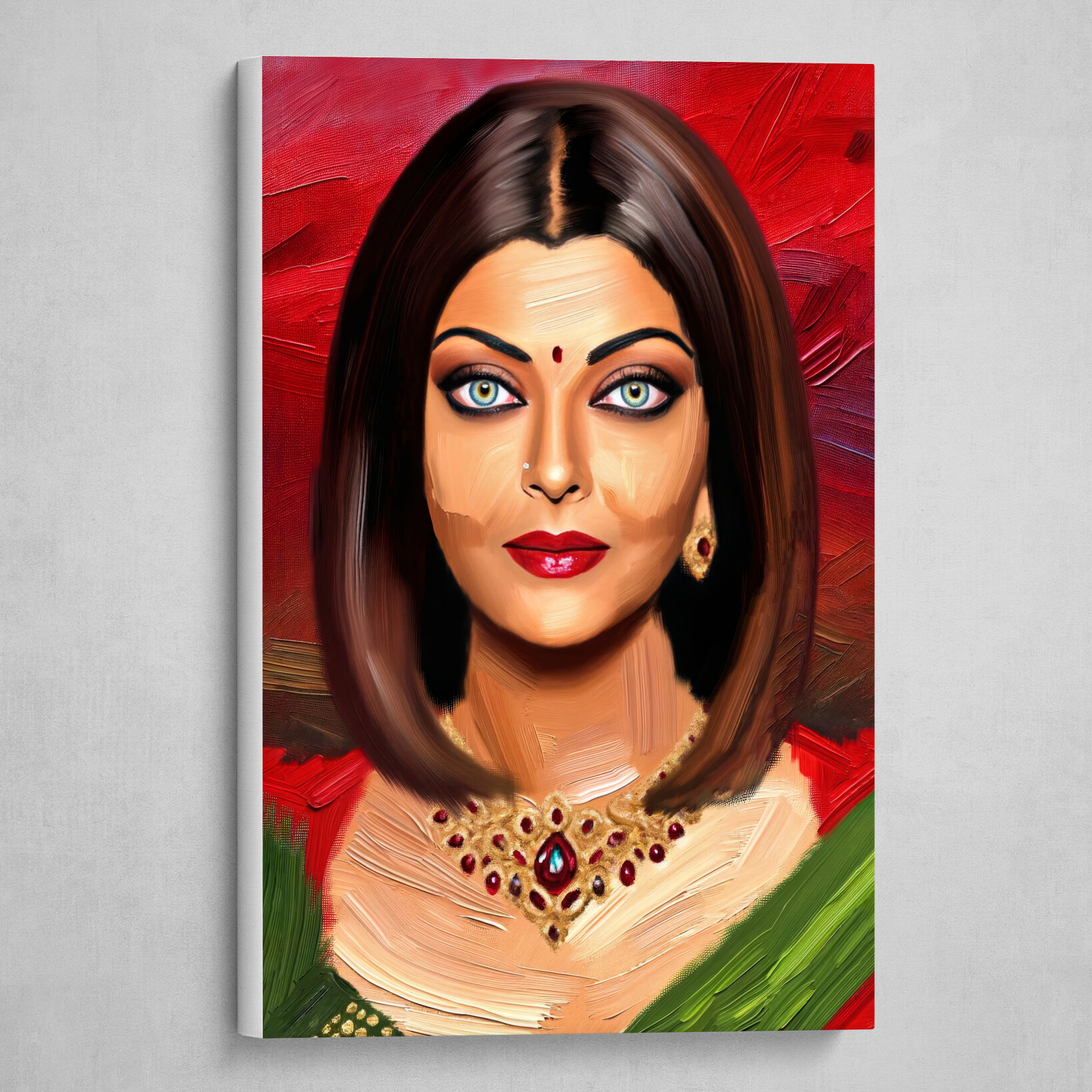The painting features Bollywood actress A. Sheree Wright depicted face-on with vibrant, expressive details. Her long bob, hitting her shoulders, is rendered in dark brown and black hues, accented with white streaks for a glossy effect. She has blue, smoky-eye makeup enhancing her bright eyes, thin eyebrows, and wears striking red lipstick. Between her eyebrows, a distinctive small red dot captures attention. Her ensemble includes a prominent gold necklace adorned with red gems and a matching ear showing a red earring, complemented by a brooch featuring a similar red ruby. The background is predominantly red, interspersed with purple and orange streaks, adding depth through textured, thick strokes characteristic of oil painting. The entire composition is set against a gray wall, highlighting the rich color palette and intricate details of the painting.